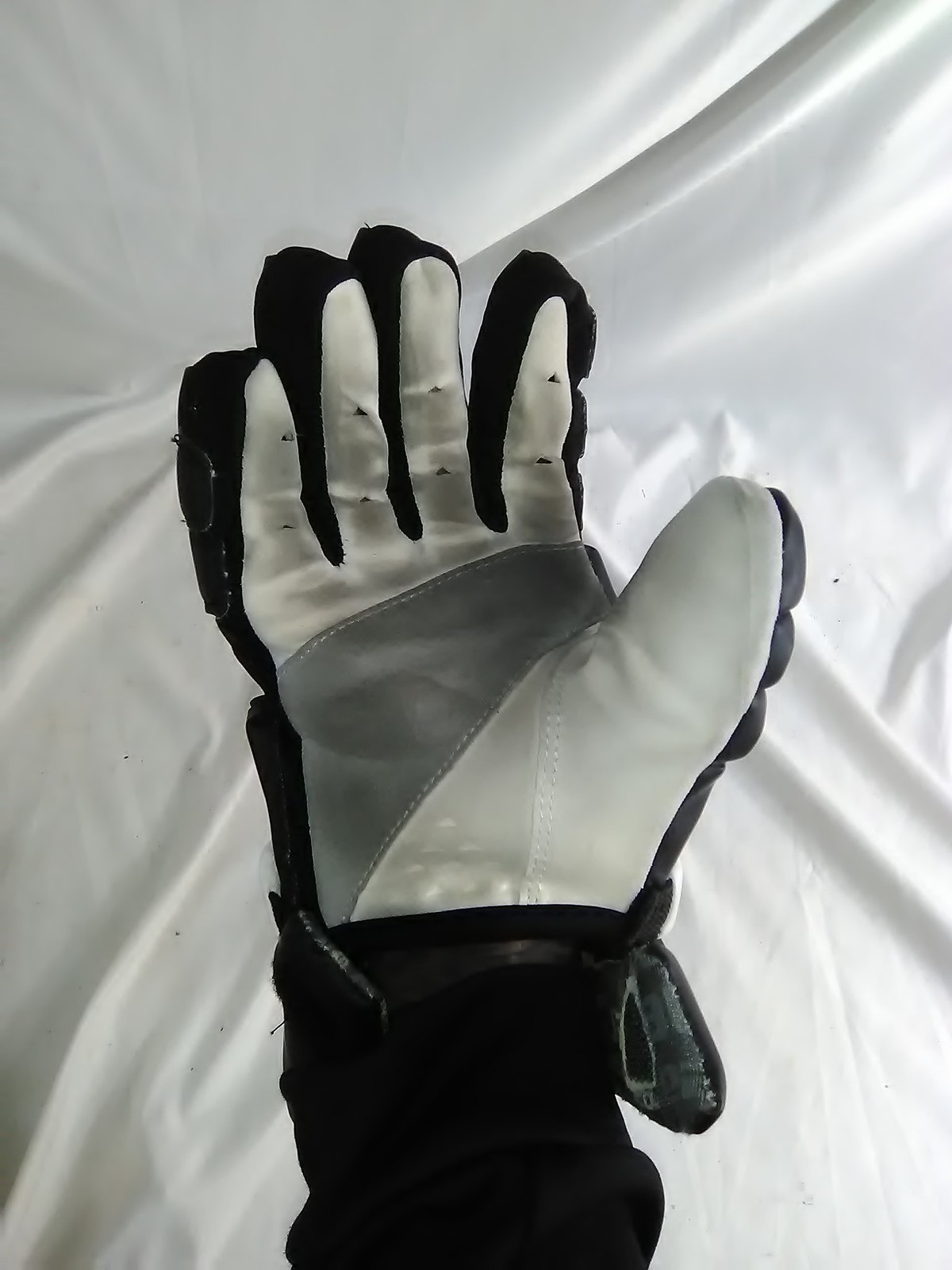This close-up photo features the underside of a high-quality right-handed glove, possibly designed for motorcycling or motocross sports. The glove is adorned in black, white, and gray tones; it features white fingers with black outlining, a gray leather section across the palm, and a black wrist strap for adjustment. The glove is resting palm-up on a crumpled white satin sheet that varies in patterns of white, light gray, and dark gray. The dimly lit image, which lacks any text or date, suggests that the glove is likely empty, although it's not possible to see beyond the wrist to confirm. The glove's padding and overall design indicate it is both warm and protective, ideal for rigorous activity requiring flexibility and durability.